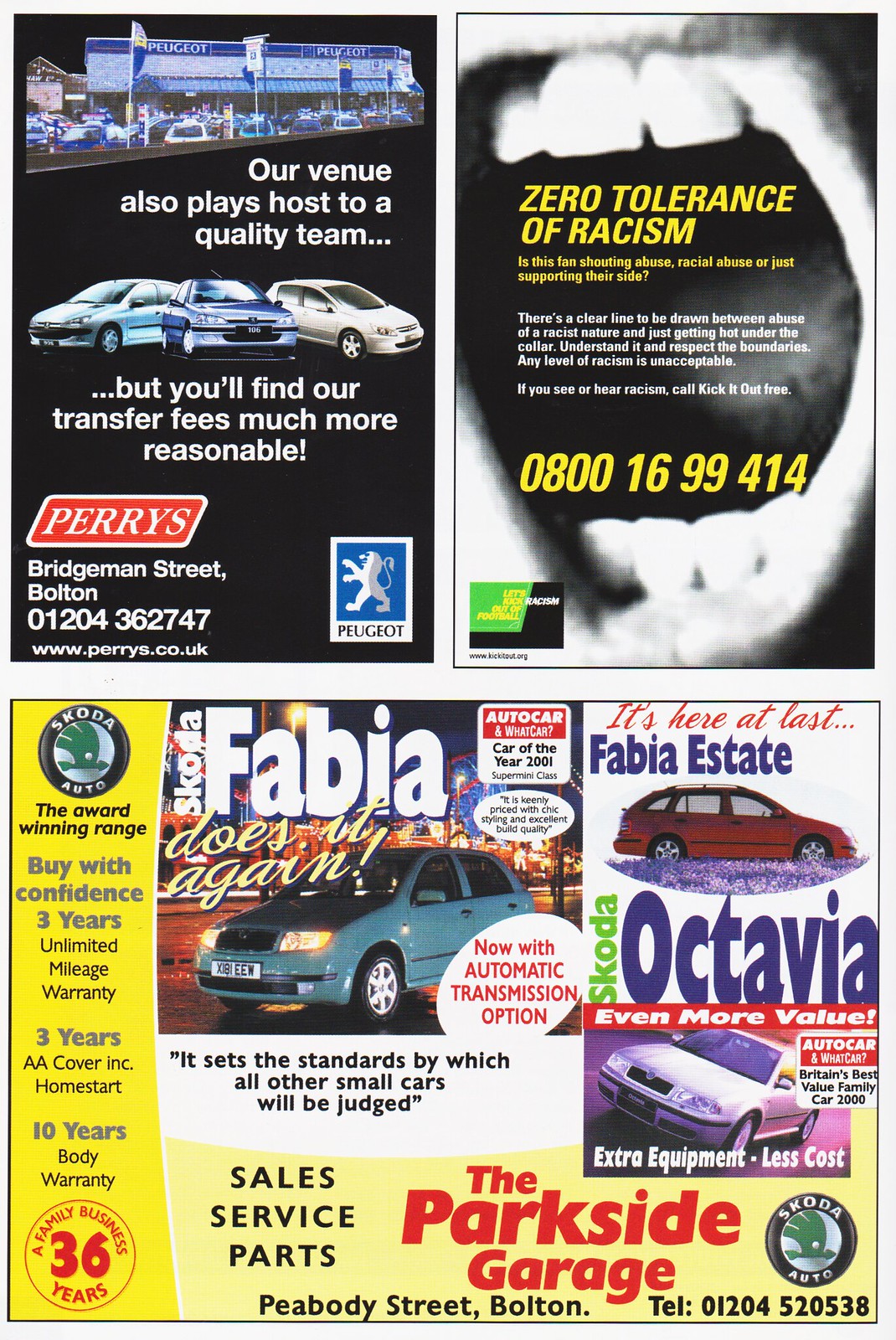The image depicts a page filled with three distinct advertisements from a marketing magazine. The top left advertisement promotes an automobile dealership, showcasing three cars alongside a message stating, "Our venue also plays host to a quality team, but you'll find our transfer fees much more reasonable." Shifting to the top right, there is an anti-racism ad that highlights a significant message: "Zero tolerance of racism. Is this fan shouting abuse, racial abuse, or just supporting their side? There's a clear line to be drawn between abuse of a racist nature and just getting hot under the collar. Understand and respect the boundaries. Any level of racism is unacceptable. If you see or hear racism, call Kick It Out for free at 0800-1699-414." Finally, the bottom half of the page features another car dealership advertisement for Parkside Garage, emphasizing vehicles like the Fabia and Octavia with slogans such as "Fabia does it again" and "Even more value, extra equipment, less cost." Additionally, it boasts about services like a three-year unlimited mileage warranty and 10-year body warranty, listing the dealership details at Peabody Street, Bolton, with a contact number 012-04-520-538. The colors used across the page include black, white, various shades of gray, blue, yellow, green, purple, and pink, creating a visually spaced and easy-to-read layout that suggests this is an advertising spread from a magazine.